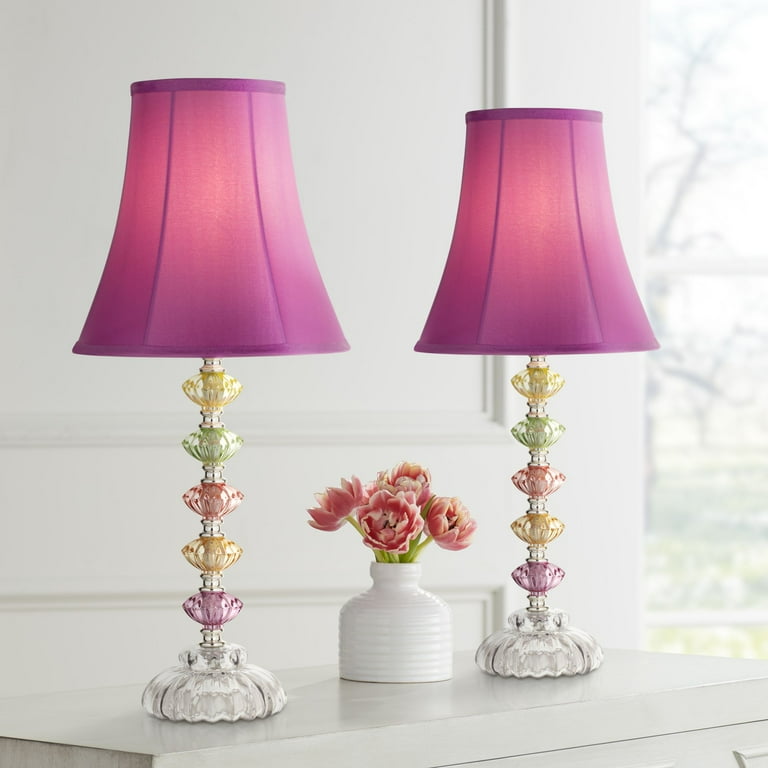The photograph showcases two identical contemporary tabletop lamps with magenta bell-shaped lampshades, positioned side by side on a table in front of a white wall. Each lamp features a base made of clear crystal adorned with colorful knobs in shades of purple, gold, orange, green, and yellow. Centered between the two lamps is a white vase containing four reddish flowers, adding a touch of natural elegance to the arrangement.